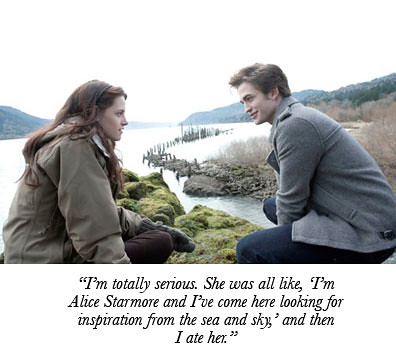The image depicts a scene that resembles one from the "Twilight" vampire trilogy. It features two characters sitting on a mossy, grassy rock by the bank of a large body of water, with a dilapidated dock extending into the water. The backdrop includes imposing mountains and an overexposed, bright white sky, indicating a daytime outdoor setting. 

On the right side sits a male character with short brown hair, wearing a gray jacket and dark blue pants. On the left side is a young woman with long reddish-brown hair, dressed in an olive green jacket and brown pants, and she is notably wearing gloves. Both characters are looking at each other.

At the bottom of the image, in quoted, italicized serif font, the text reads, "I'm totally serious. She was all like, 'I'm Alice Starmore and I've come here looking for inspiration from the sea and sky,' and then I ate her."